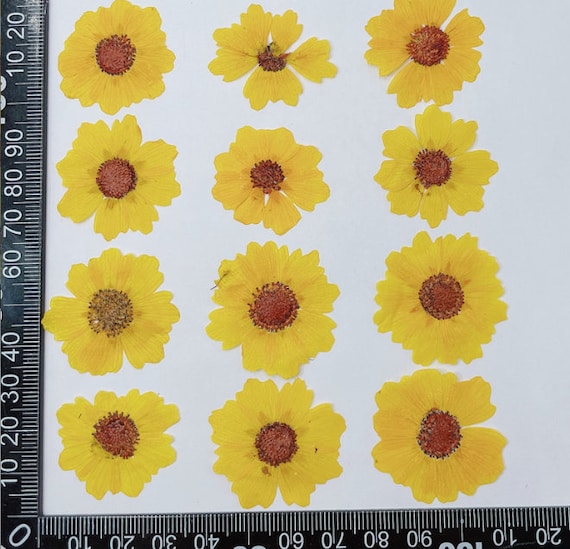The image depicts a piece of white fabric adorned with a repetitive daisy pattern arranged in a grid of four rows and three columns. Each daisy features yellow petals and centers that vary in shades of red and brown, described as deep burnt orange. Flanking the fabric are two black rulers with white markings: one aligned vertically along the left edge, and another horizontally along the bottom edge, although upside down. These rulers, which bear sequential measurements in increments of 10 up to 100 and beyond, help hold the fabric in place for precise measurement and cutting, possibly for crafting clothing or other fabric-based items.